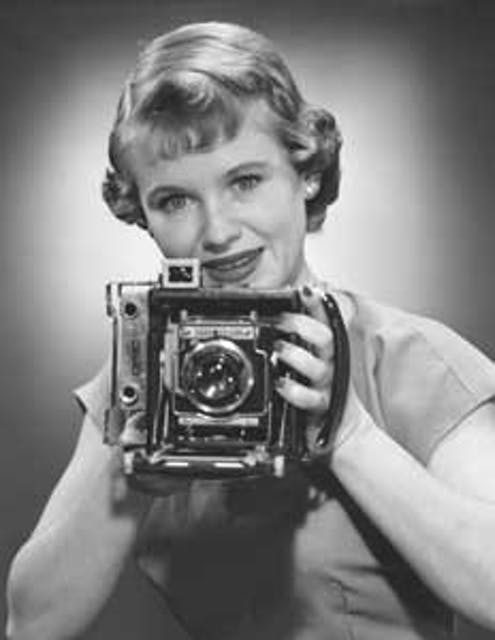This black and white vintage photo captures a relatively young woman with a slightly curly, short haircut that just covers her ears. She is holding a large, old-fashioned, boxy camera in both hands at chin level. The camera features a square viewer and a circular lens, indicating its age. The woman gazes directly at the viewer with bright eyes, a nervous smile, and her mouth slightly open, revealing a mole on her chin. She is dressed in a solid-colored, short-sleeved dress, and her nails are painted dark, matching her earrings. The background is a simple gradient that transitions from white near her face to dark gray towards the edges, enhancing the vintage feel of the photograph.